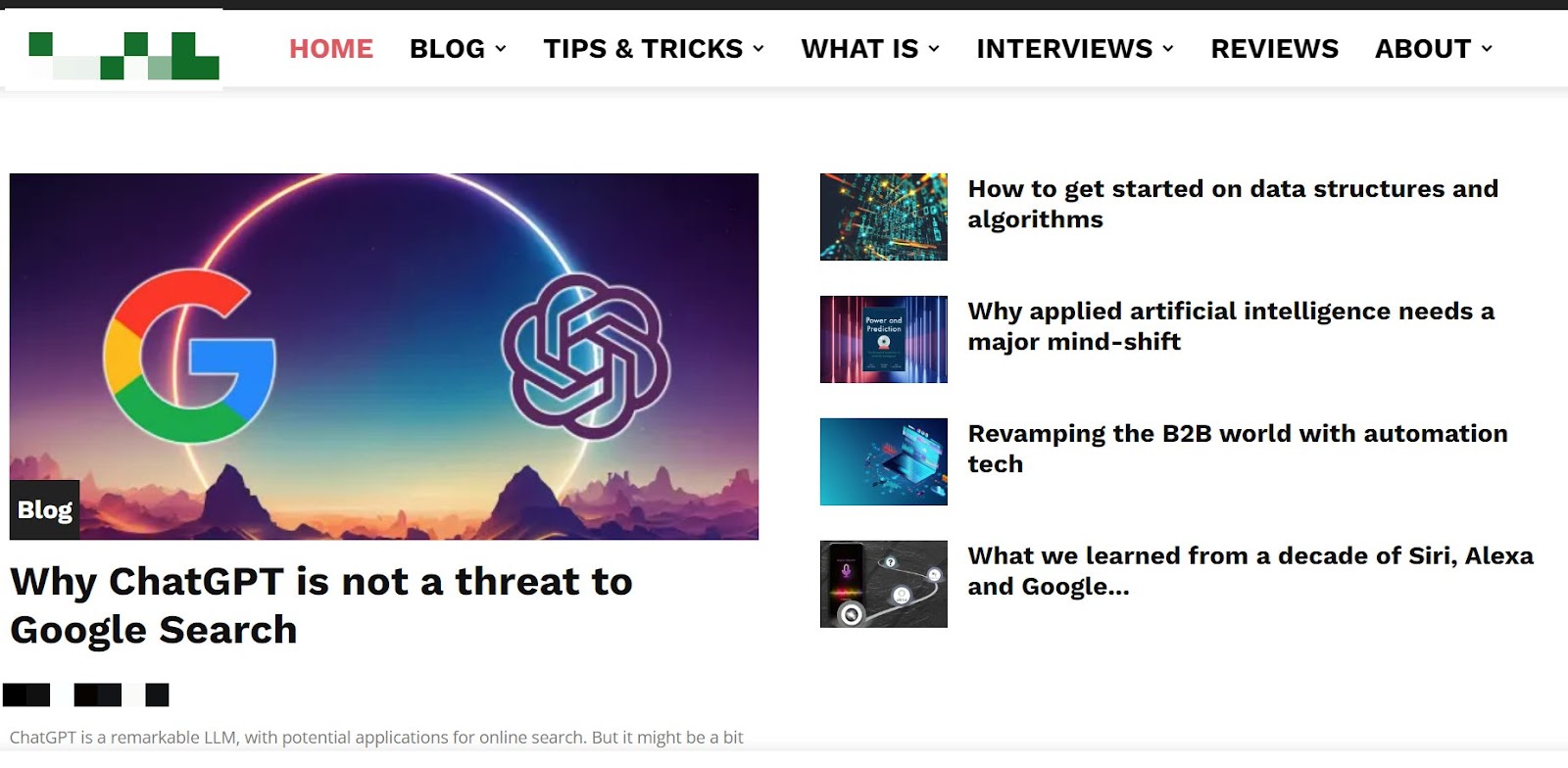In the image, there is a series of colored and white squares arranged as follows: a green square, a white square, another white square, a green square, a green square, a white square, a gray square, a green square, and three consecutive green squares. Below this sequence, there is a white bar with the word "Home" written in red text, followed by "Blog" in black. The navigation also includes "Tips and Tricks," "Interviews," "Reviews," and "About." The letter "G" appears prominently, and the sky in the background is depicted in a striking purple color. There is also a ring visible in the scene. Featured articles include "How to Get Started on Data Structures and Algorithms," "Why Applied Artificial Intelligence Needs a Major Mind Shift," "Revamping the B2B World with Automation Tech," and "What We Learned from a Decade of Siri, Alexa, and Google." The entire layout sits on a white background and appears to be part of a tech news website, which also features an article titled "Why Chat GPT is Not a Threat to Google Search."